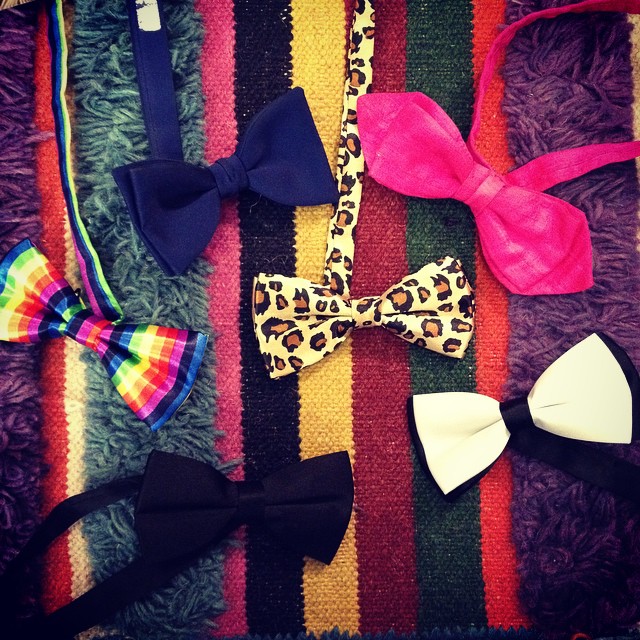This close-up photograph showcases an assortment of uniquely designed bow ties, meticulously laid out on a strikingly colorful, multi-textured background. The backdrop begins with a stripe of purple carpet, followed by a red stripe, a tan stripe, a section of another fabric, then dark gray carpet, and continues with stripes of pink, black, yellow, maroon, dark green, another red, and ends with a purple stripe. The bow ties, arranged with precision, feature a dark blue bow, a vibrant hot pink bow, and a striking rainbow-colored bow with shades transitioning through blue, green, yellow, orange, red, purple, and dark blue. Additionally, there's a bold leopard print bow, a pristine white bow edged in black, and a traditional black bow. Though these bow ties are small, perhaps indicative of women's fashion, the focus remains sharply on their vivid patterns and varied materials, creating a visually engaging composition against the textured, colorful surface.